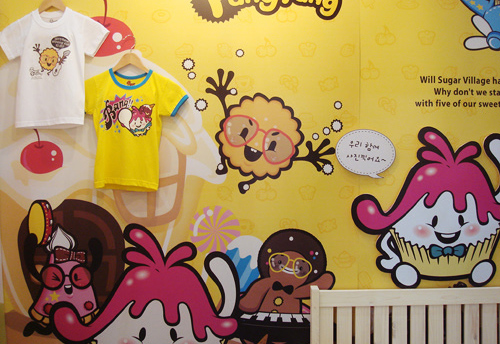The image depicts a vibrant, cartoon-themed display, set against a cheerful yellow background adorned with tiny illustrations of fruits and candies. Various animated food characters are painted on the wall. Prominent among them is a cookie with sunglasses, and a pink-haired cupcake in a yellow liner wearing a bow tie. Below, a gingerbread man with a brown hat and yellow sunglasses plays an electric piano, waving with one hand. In the bottom left corner, a small gumdrop-shaped character with round black sunglasses adds to the playful scene. Two children’s t-shirts hang on the upper left: one white, featuring the cookie character, and another yellow, highlighting the cupcake character. The upper wall has text that reads, "Will Sugar Village HA Why Don't We Stay with Five of Our Sweet." In the lower right corner, there appears to be part of a crib or small fence. The detailed illustration captures a whimsical and delightful setting, perfect for a child’s room or a playful display.